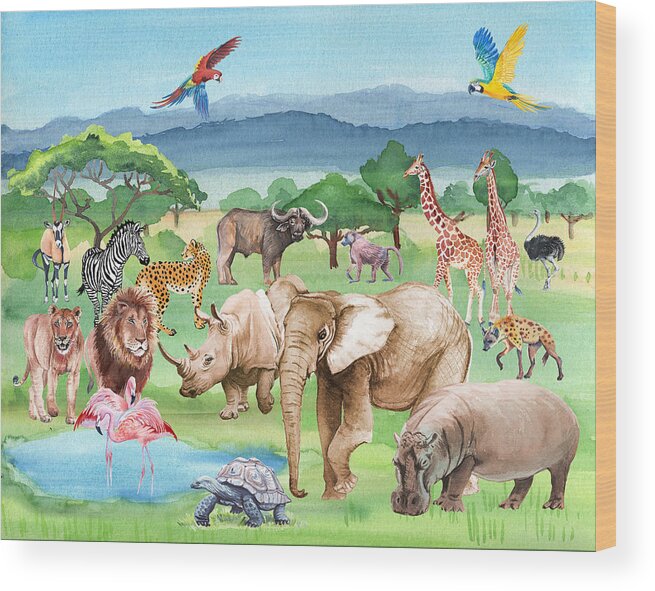This captivating wildlife painting, set against the plains-like landscape with numerous trees, features a light blue sky and two vibrant macaws, a red one to the left and a yellow one to the right, each adorned with blue and yellow feathers. Background elements include light and dark blue mountains and a variety of African-like trees, some bushy and some tall and spread out.

The scene showcases a diverse array of animals densely grouped together in a vivid green field. In the bottom right appears a smaller hippopotamus, adjacent to a large elephant, with a rhinoceros close by, near a male and female lion. There is a pond to the left of these, where two flamingos wade, with a large tortoise in the foreground. Central to the painting, a cheetah, hyena, and zebra are depicted, with the zebra directly observing the cheetah. An antelope, water buffalo, and ostrich are also present, alongside two giraffes and a monkey or gibbon. The meticulous detail extends to elements like the animals’ postures and interactions, creating a rich and dynamic tableau on canvas.